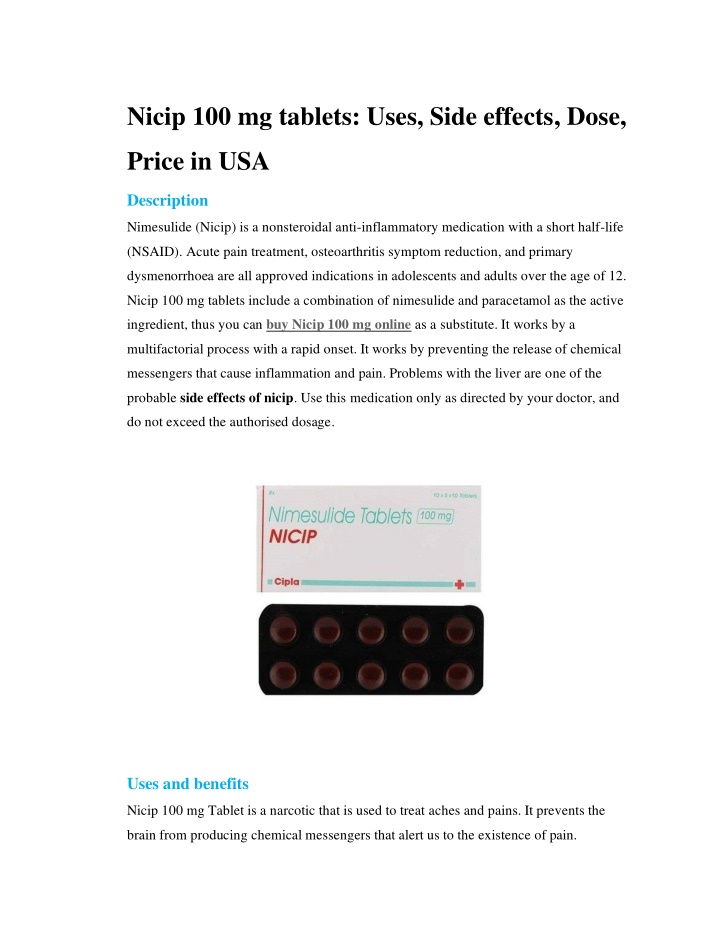The image has a white-to-black gradient background. At the top, the text in black reads "NICIP 100 mg tablets." Following that, in black text, the image provides information on side effects, dosage, pricing, and its availability in the USA. 

In light blue text, the heading "Description" appears, followed by more detailed information in black. It states that NICIP contains the active ingredients nimesulide (a non-steroidal anti-inflammatory drug or NSAID with a short half-life) and paracetamol. NICIP is indicated for the treatment of acute pain, reduction of symptoms in osteoarthritis, and primary dysmenorrhea in adolescents aged 12 and above. 

The tablets can be purchased online, as indicated by the underlined text: "Buy NICIP 100 mg online." 

The descriptive text explains that NICIP works by a multifactorial process with a rapid onset, preventing the release of chemical messengers responsible for inflammation and pain. Users are advised to follow the prescribed dosage and consult a doctor to avoid potential side effects.

The tablet packaging is primarily white, with red accents and text indicating "10 tablets" in red and black. The information concludes with a section in blue text headed "Uses and Benefits."